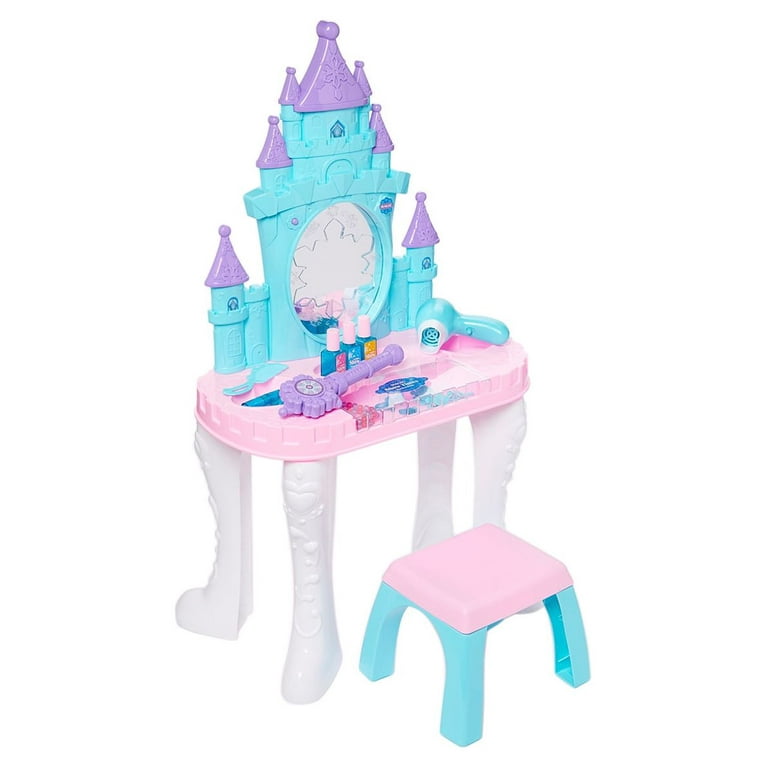The image depicts a child's princess-themed vanity set, designed primarily for little girls. The set features a petite vanity table with white legs and a pink tabletop. The back of the vanity is designed to resemble a fairytale castle, painted in shades of blue and lavender, with purple rooftops and a central mirror adorned with a snowflake pattern. Accompanying the vanity is a small bench with a pink seat and blue legs.

On the tabletop, various toy accessories are carefully arranged, including a teal hairdryer with a white tip, a teal comb, a purple hand mirror, and three bottles of nail polish in teal with colorful labels and pink caps. Additionally, there is an unidentifiable purple scepter-like object. The entire set is presented against a plain white background, suggesting it is an image intended for showcasing the product, perhaps on a retail site.